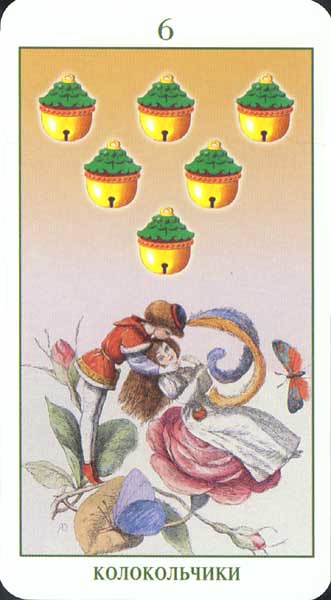A vertically oriented image with Russian writing at the bottom is held in place by corner holders. At the top center, there is a green number 6. Below this number, a stylized green outline depicts six bells arranged in a triangle with three on top, two in the middle, and one at the bottom. Beneath the bells, a woman in a flowing white dress sits gracefully on a giant red rose. In front of her hovers a delicate butterfly. Behind her, a gentleman with red hair and wearing a hat adorned with large feathers places his arms around her shoulders. He is dressed in a short-sleeved red jacket over a white shirt, complemented by white leggings and red shoes. The gentleman stands on the branch of the rosebush, with a giant rosebud behind him adding a whimsical touch to the scene.